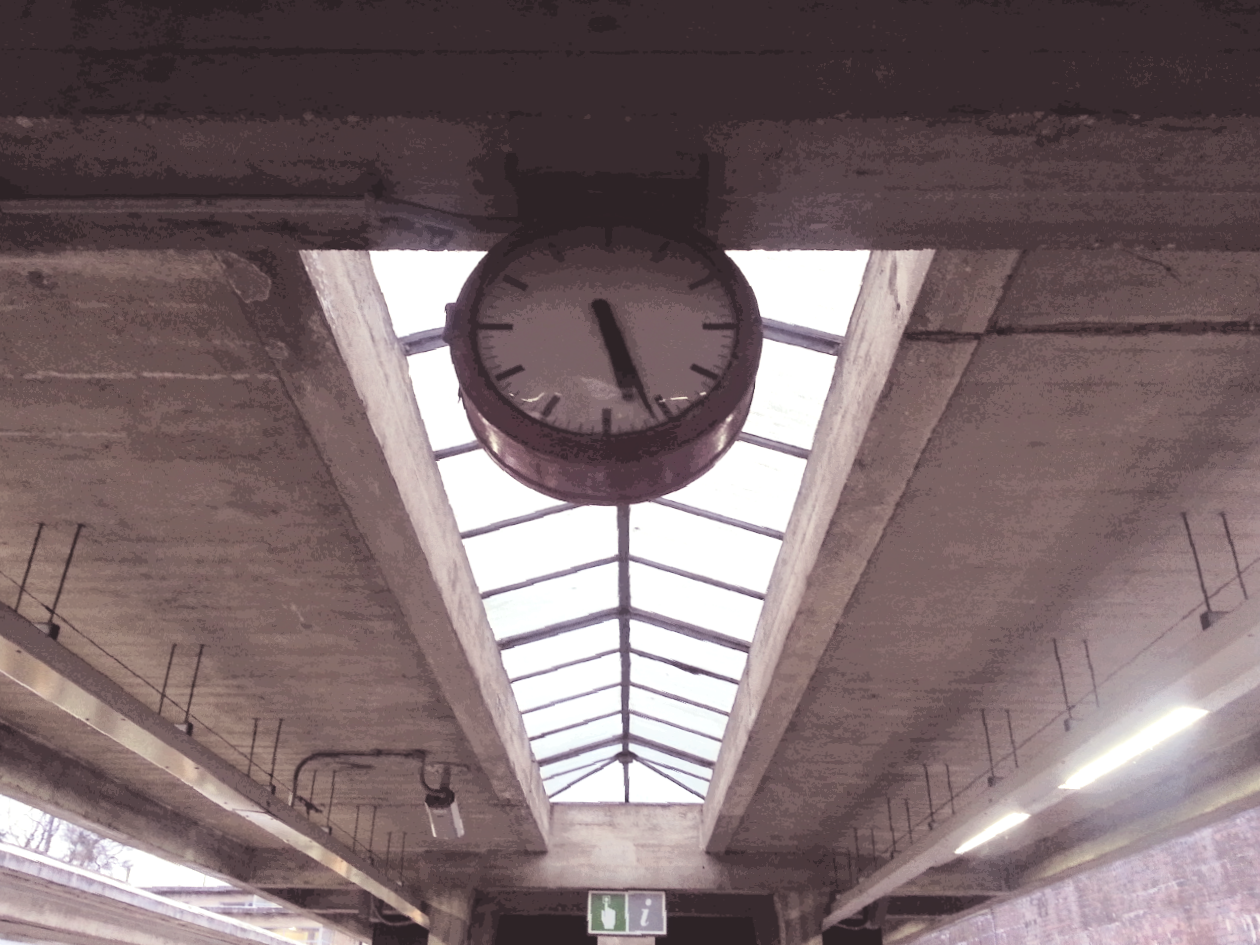The photograph captures a clock suspended from the ceiling of an industrial-style building. The ceiling is made of gray stone and features an opening with metal arched windows running down the center, resembling a skylight that illuminates the interior space. Along the gray stone ceiling, black metal fixtures extend downward, supporting fluorescent tube lights encased in metallic housings. The clock itself is circular with a gray frame and a white face, notably lacking numbers. The clock hands indicate the time as 5:26.